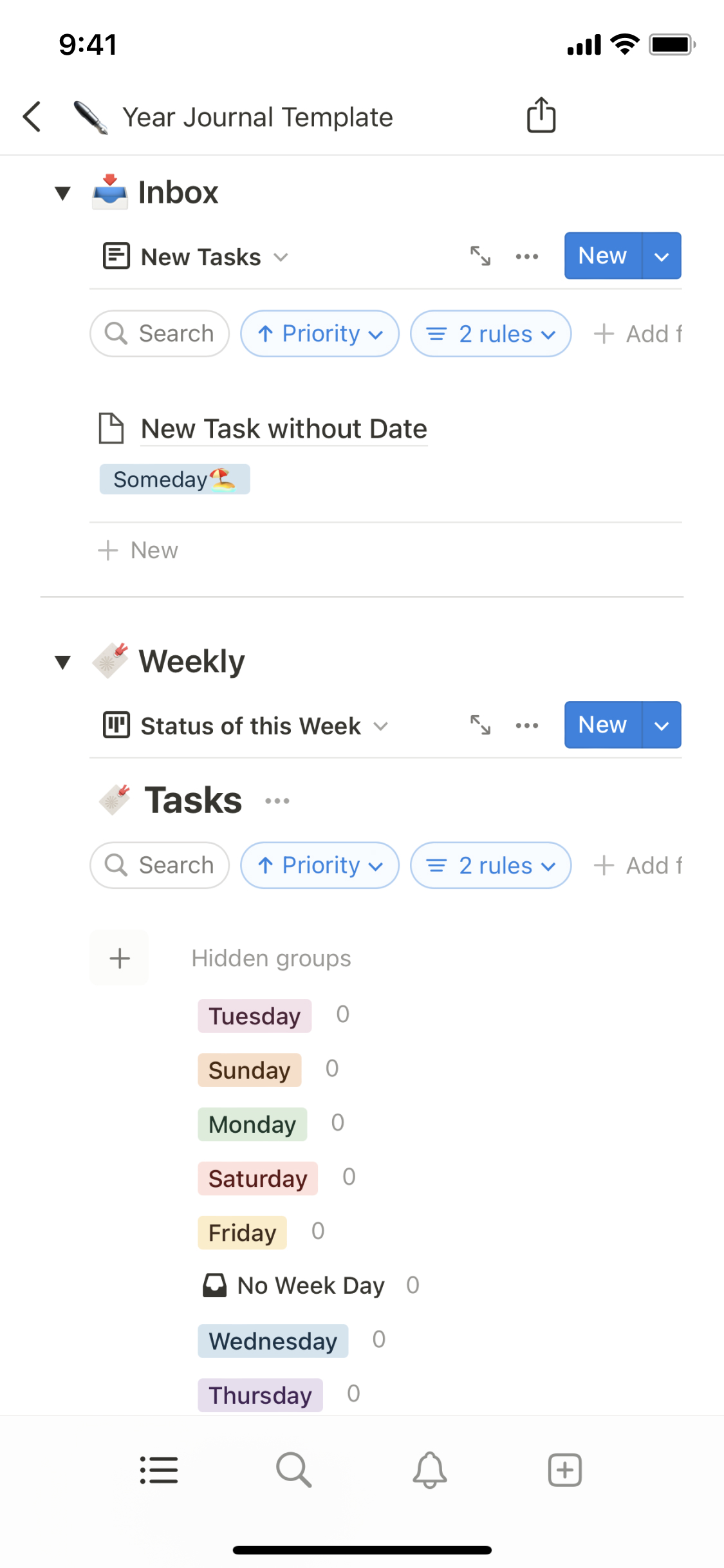**Caption:**

The image depicts a smartphone screen at 9:41 (no indication of AM or PM). The device shows full signal bars, Wi-Fi enabled, and a fully charged battery. At the top left, a back arrow suggests the ability to navigate backwards.

At the center of the screen is an image of a fountain pen next to text that reads "Year Journal Template" with an upload option available. Below it, "Inbox" is visible followed by an icon resembling a paper with writing, labeled "New Tasks." The word "New" is displayed in blue next to a drop-down arrow for additional options.

Further down, there are fields labeled "Search," "Priority," and "Two Rules," accompanied by an "Add One" option. Following that, the screen shows a blank, folded piece of paper icon labeled "New Task Without Date," with a sub-label "Someday" featuring an umbrella on a beach.

Moreover, there are sections for "Weekly," "Status of the Week," and "Tasks." Each day of the week—Tuesday, Sunday, Monday, Saturday, and Friday—shows zero tasks, and similarly, Wednesday and Thursday also indicate zero tasks.